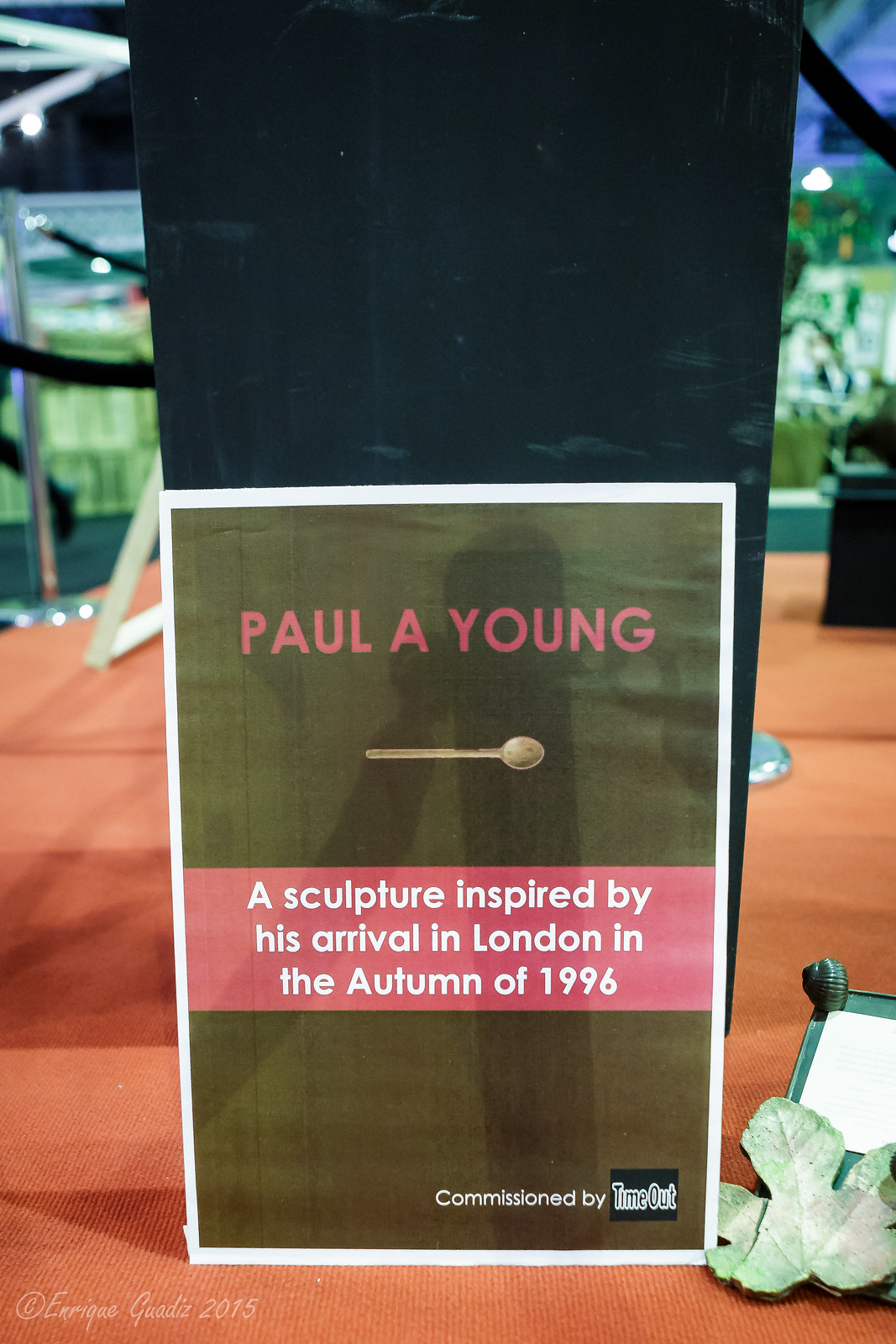This photograph captures an intricately designed sign prominently placed within an interior room, possibly a museum or showroom showcasing the work of Paul A. Young. The sign features a vibrant red text against a green background, reading "Paul A. Young," and is accompanied by the image of a simple spoon. Beneath the name, in a similarly colored red box, the text states, "A sculpture inspired by his arrival in London in the autumn of 1996." At the bottom, it reads, "Commissioned by Timeout" in black text outlined in white against a green backdrop. The sign is affixed near a dark-colored pillar or column anchored to a floor covered in a light orange or burnt orange carpet. Additionally, a part of the black sculpture, which seems to be broken or incomplete, is visible behind the sign. The scene includes a divider post with a rope to the left, further suggesting a curated space for showcasing artworks. The overall setting is meticulously arranged to emphasize Paul A. Young's work and the narrative of his inspiration from arriving in London.